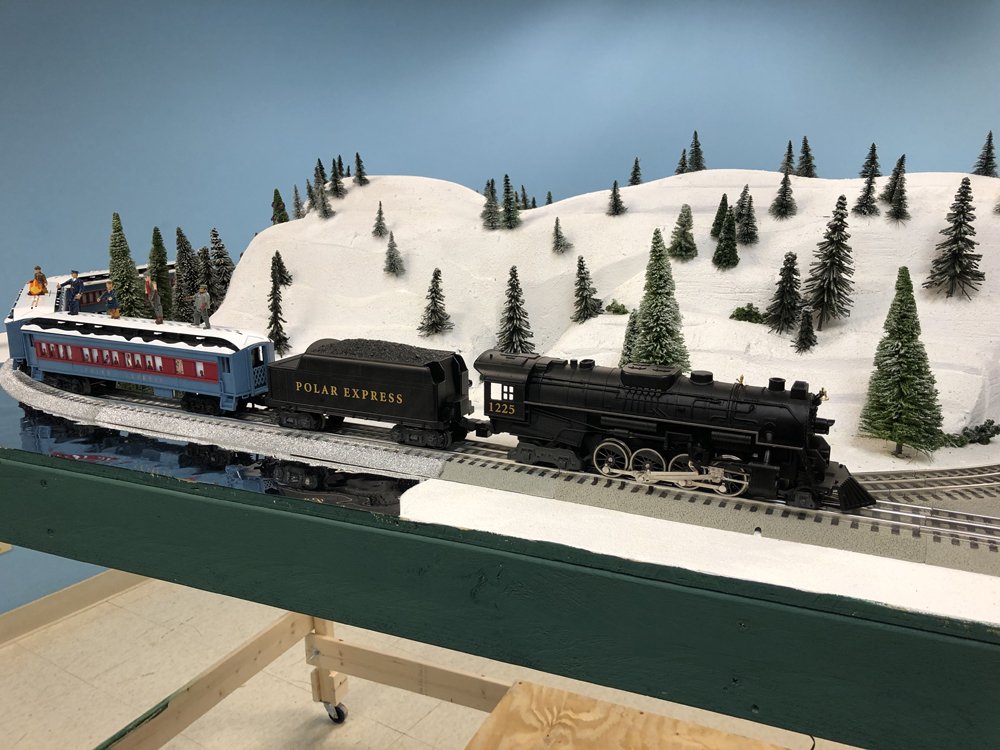The image captures a detailed miniature train set depicting a scene from the Polar Express on a movable table. The photo features a vibrant blue sky backdrop at the top, transitioning to a central landscape filled with mountainous, snow-covered rolling hills and dotted with green pine trees. A prominent brownish railroad track circles the snowy mountains. The train is a locomotive set consisting of a blue engine with red-trimmed windows, followed by a coal car emblazoned with "Polar Express" in gold letters, and three black passenger carts. The train set rests on a green track, positioned on a gray, snow-like surface with yellowish-brown wooden beams visible underneath, supporting the entire display.